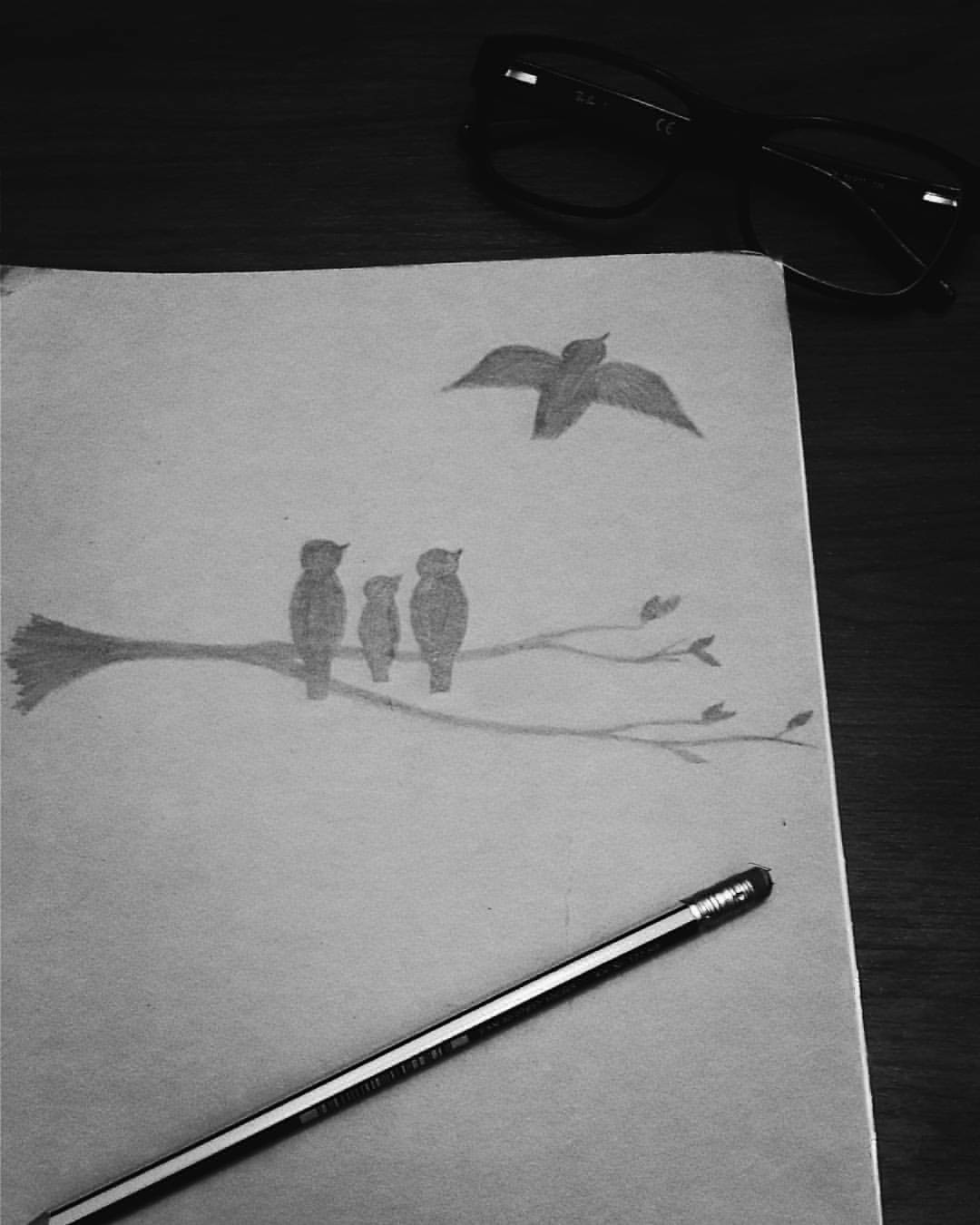A captivating pencil sketch dominates the page of a sketchbook that lies open on a dark tabletop, creating a striking contrast. The photograph captures this monochrome scene from an angle that frames the top and left side of the book. Near the lower left corner of the image, a pair of glasses rests subtly; though almost swallowed by the darkness, their shape is still discernible. Positioned horizontally across the bottom of the sketchbook page is a sleek silver pencil, adding a touch of metallic elegance to the composition.

The sketch itself portrays a serene yet dynamic scene of avian life. A trio of birds is perched gracefully on a tree branch; the larger two birds occupy the uppermost portions of two diverging secondary branches, while a smaller bird shares the space with them. Delicately rendered leaves sprout from the tips of thinner twigs, completing the tranquil tree motif. The focal point of the sketch is the fourth bird in mid-flight, departing from the ensemble of perched birds. Every element, from the birds to the foliage, is intricately detailed in various shades of gray, emphasizing the skill and precision of the pencil work.